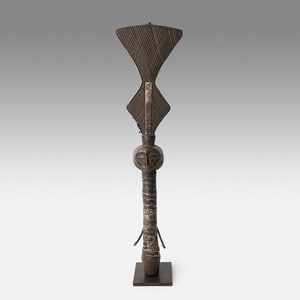This tall, hand-carved wooden statue, rendered in dark brown hues, exudes the intricate craftsmanship of African artistry. Its form begins with an upside-down triangle shape at the top, gracefully transitioning into a diamond shape that encompasses the head of the figure. The head is rounded, featuring a striking facial expression where one eye appears to be open and the other closed, giving it a lifelike, blinking appearance. This piece, embodying the essence of traditional African artifacts, would feel at home displayed in a museum or as part of an exquisite personal collection.